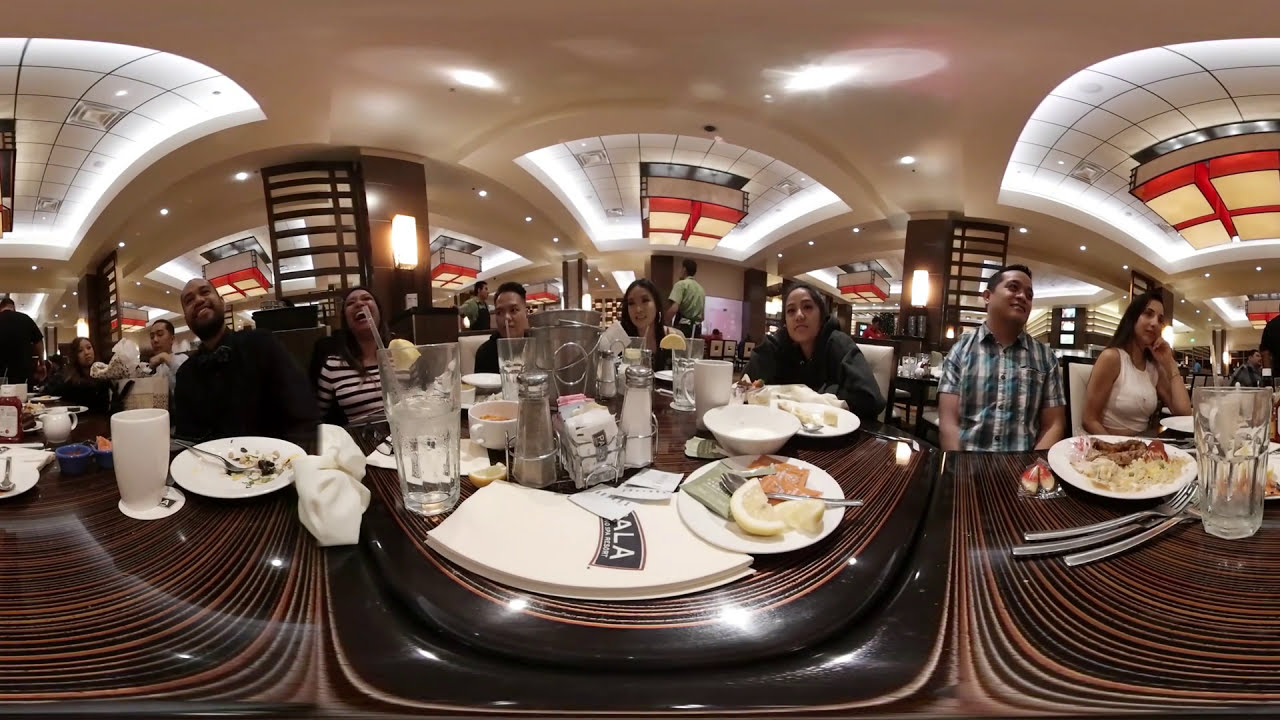In this detailed panoramic fisheye image, we see a bustling indoor restaurant setting with a series of connected brown dining tables adorned with plates of food, white napkins, water glasses, and condiments like salt and pepper. The convex image, which creates a rounded effect on the ceiling and gives a wide, almost 360-degree view, captures multiple people enjoying their meals. At the central table, we see four Asian individuals—a man and three women—surrounded by various dishes possibly including meat, pasta, and a lemon slice. There are also four people on the left and three on the right, with some seemingly engaged in conversation and laughter, while others appear more subdued, continuing their meals. A notable man on the left handles a white coffee cup with an empty plate. Among the food items visible are a fortune cookie, suggesting Chinese cuisine. Overhead, the roof features distinct lighting fixtures with red outlines, adding to the restaurant's warm ambiance. In the background, a server in a green shirt attends to other diners, enhancing the lively and inviting atmosphere of the scene.